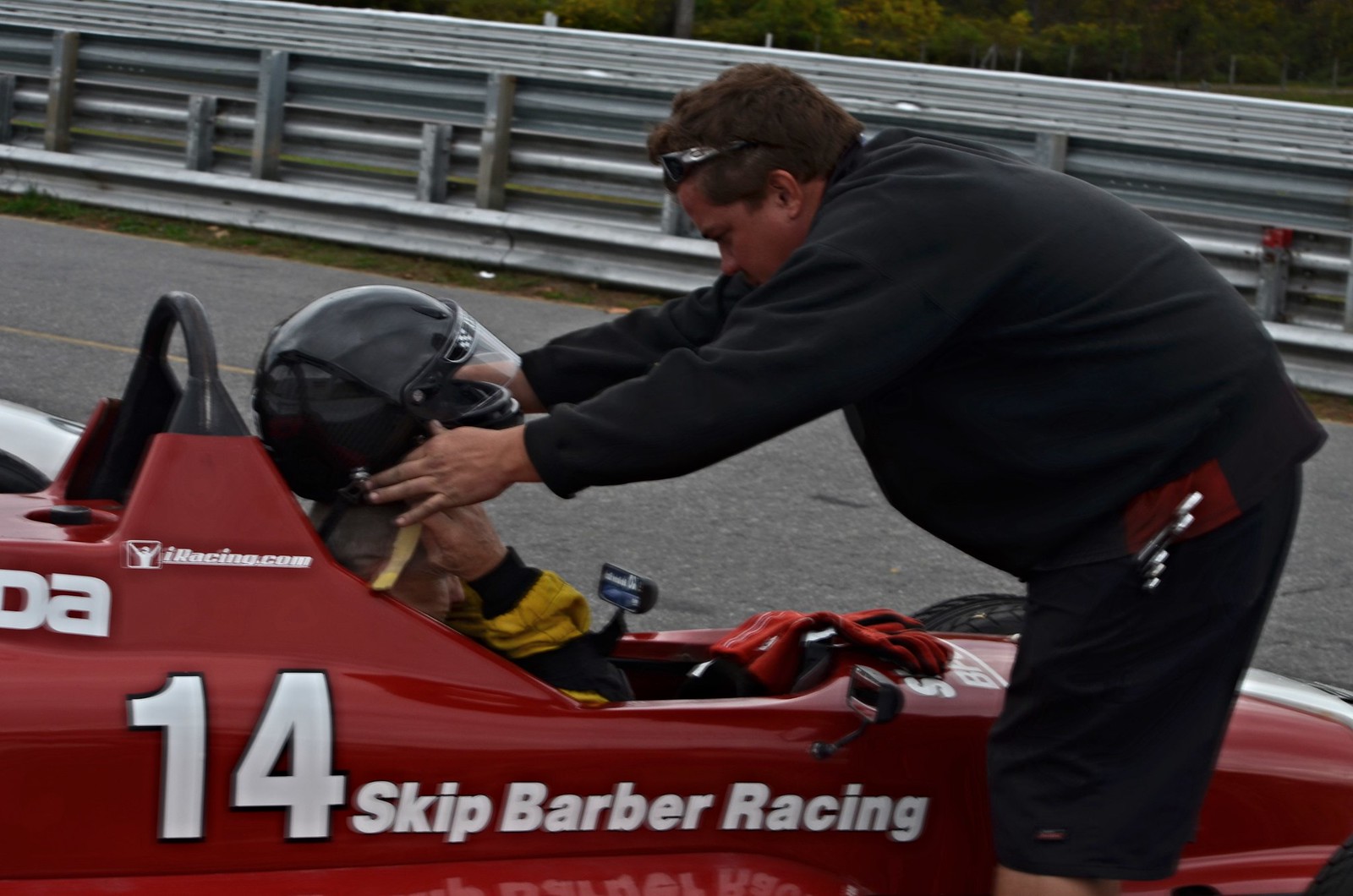The image depicts a detailed scene at a racetrack featuring a red Formula racing car marked with the number 14, "Skip Barber Racing," and "iRacing.com," along with a partial Mazda logo. The car is an open-wheeled, dragster-like race car parked on the track's grey pavement, with a metal guardrail and trees visible in the background.

A white man with brown hair, wearing a black long-sleeve shirt, black shorts, and sunglasses pushed up on his head, leans over the driver’s seat. He is adjusting a black helmet on the head of the seated driver, who is also seen securing the helmet's chin strap. The driver's shirt features gold and black colors, and the Formula car's steering wheel is not yet installed, indicating that preparations are still underway. The scene captures the moment just before the driver, appearing focused and ready, positions himself for the race.